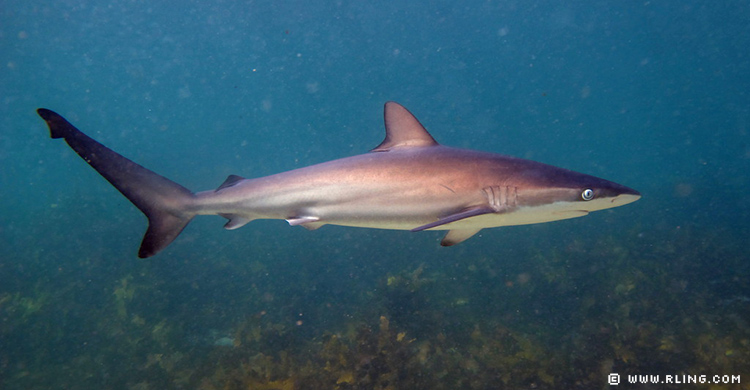This is a detailed, horizontal, underwater photograph predominantly featuring a small shark swimming towards the right side of the frame. The shark has a very light gray to grayish-brown coloring with a white underbelly, a distinctive short top dorsal fin, shorter side fins, and a unique tail marked by a black stripe along its backside. The scene is set in light navy blue water, with sunlight casting visible highlights on both the shark and the surrounding vegetation. The background is dense with aquatic plants, likely seaweed, and possibly plankton or other small sea particles floating in the scene. The overall atmosphere is somewhat dark with cloudy water. A small fish can be seen swimming near the shark. In the bottom right corner of the photo, there is a copyright symbol followed by the website address "www.rling.com," indicating that this could be a professionally taken image intended for use on a website or publication about marine life.